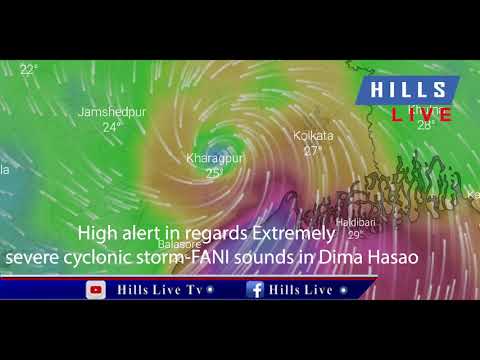This detailed screenshot captures a weather map depicting an extremely severe cyclonic storm named FANI over a region identified as Dima Hasao, possibly in Pakistan. The map, heavily color-coded with green, brown, purple, and beige areas, indicates varying degrees of moisture and storm intensity, overlaid with white wind patterns to exemplify the extensive affected area. The map’s authenticity appears altered or enhanced for visual emphasis. At the bottom, the text provides a "High alert in regards to the extremely severe cyclonic storm FANI," while the local news station’s logo, "Hills Live TV," along with a Facebook symbol, is also visible.